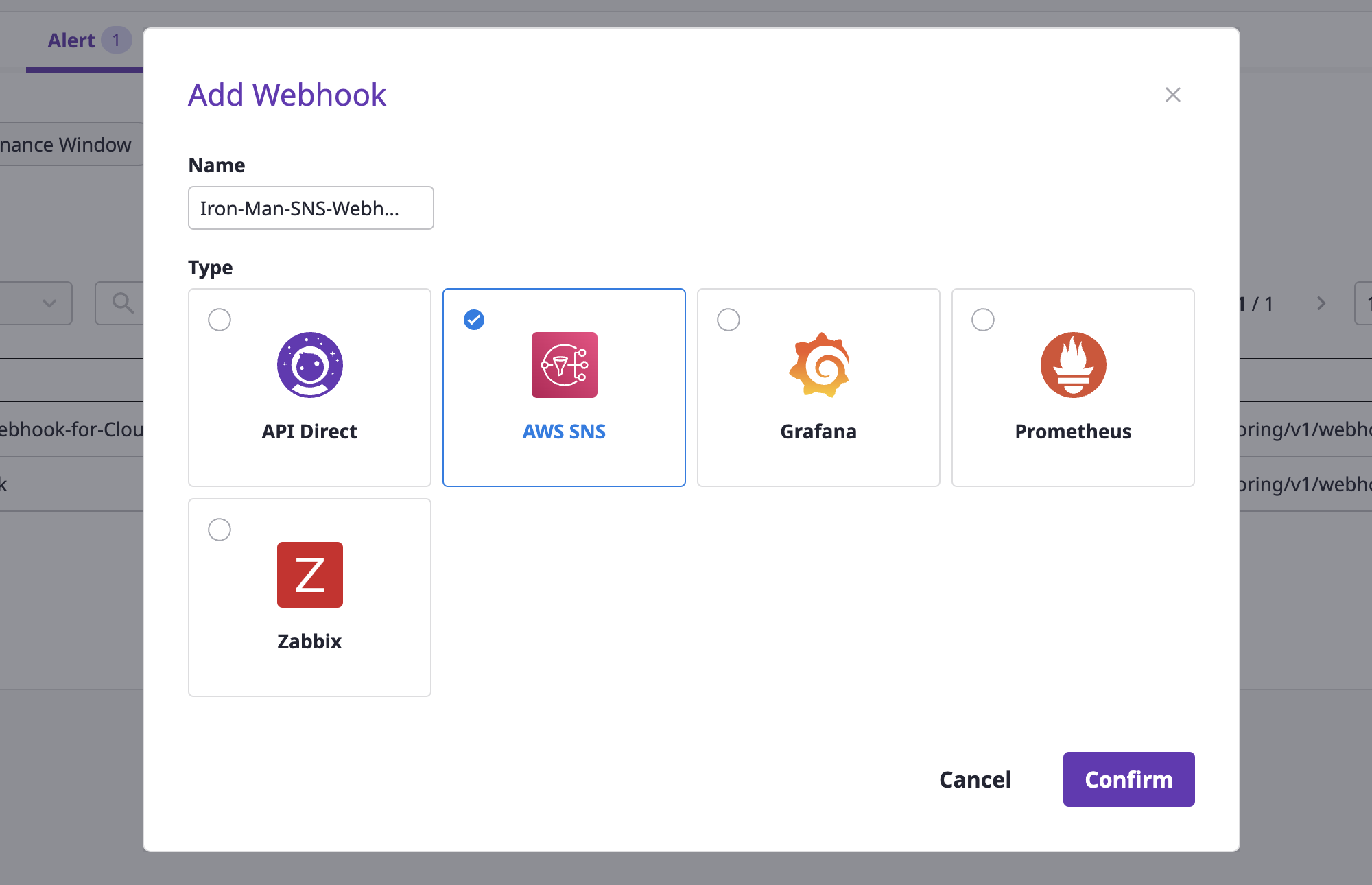This image displays a webpage interface designed for adding a webhook. At the top left corner of the interface, the text "Add Webhook" is prominently featured in a purple or indigo font. Directly below this is a text field labeled "RMSS WebH," likely for entering the webhook name. Another text field beneath this is similarly labeled "RMSS WebH," and below it is the label "Type."

The interface has four widget sections at the top and one at the bottom. In the top-left widget, there is an "API Direct" option indicated by a purple lock icon. To its right is another widget labeled "AWS SNS." The next widget, labeled "Grafana," features an icon resembling a yellow gear. Adjacent to this is the "Prometheus" widget, marked by a red circle containing a torch-like symbol.

Below this row, there is a widget for "Zabbix," represented by a red square with a white "Z" in the center. Each of these widgets is enclosed within a light gray square outline, maintaining a consistent and organized layout.